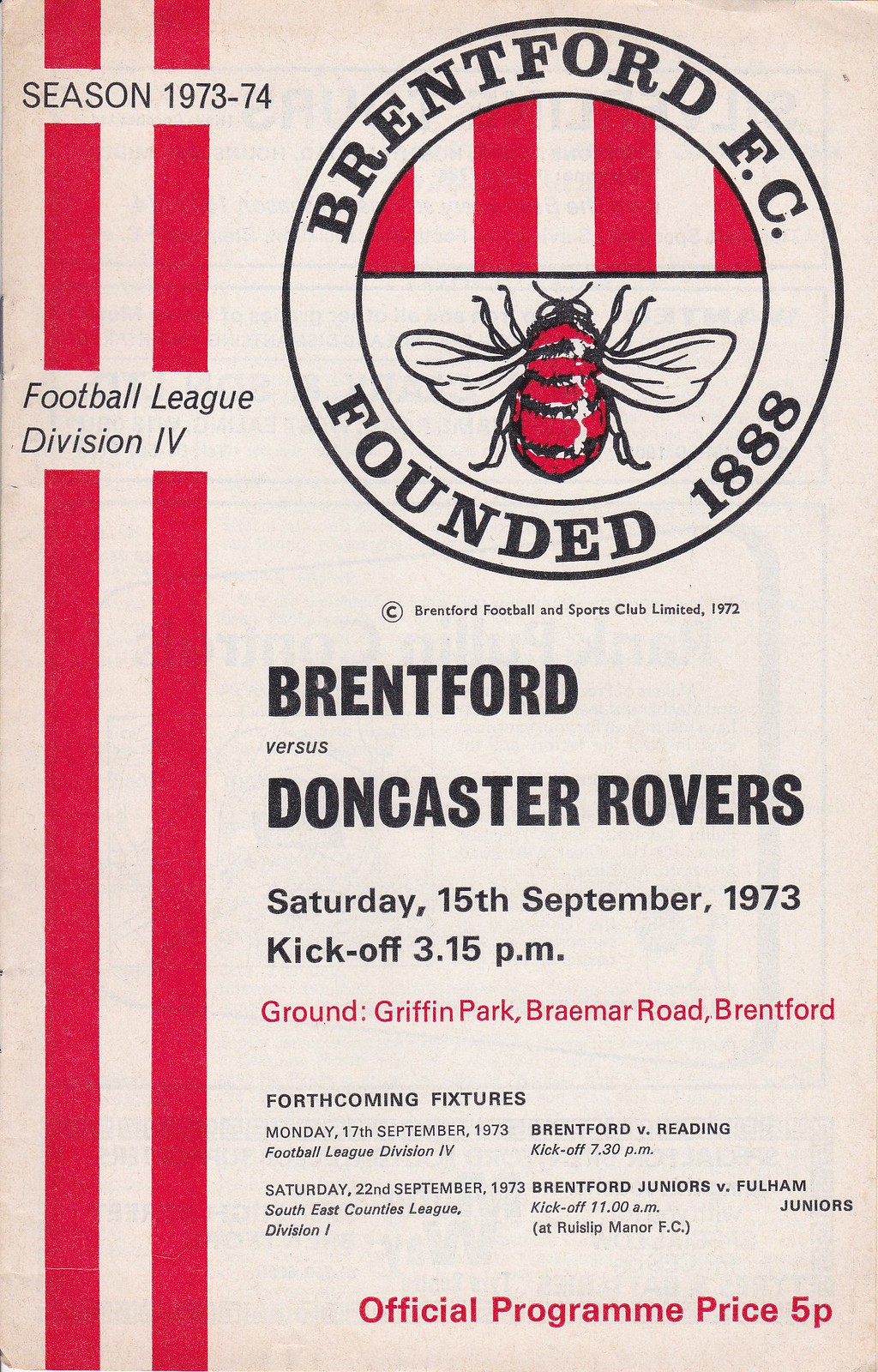This is the cover of an official game day program for a football match. The cover itself is predominantly white, featuring two thick vertical red stripes on the left side. At the top left corner, the text "Season 1973-74" is prominently displayed, with "Football League Division 4" positioned just below it, centered above the two red lines. On the top right side, there is a significant black circle with an emblem. Encircling this emblem is the text "Brentford FC founded 1888." Within the emblem, there are red and white vertical stripes on the top half, and a red bee beneath them. Below this emblem, large text reads "Brentford vs. Doncaster Rovers, Saturday 15th September 1973, kickoff 3.15 p.m., ground Griffin Park, Bramer Road, Brentford." Additionally, a section beneath this provides information on forthcoming fixtures, with smaller red text at the bottom right stating, "Official Program, price 5p."